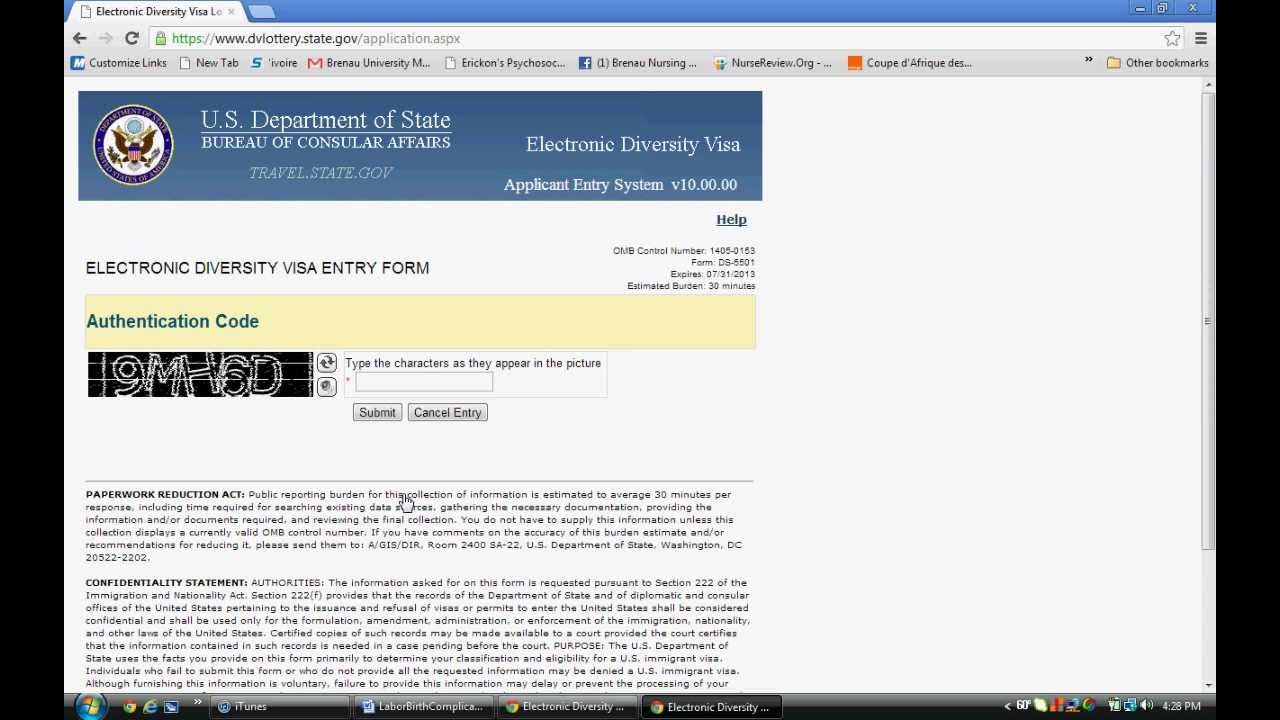This image is a screenshot of a computer desktop running Windows, as evidenced by the taskbar located at the bottom of the screen. On the far left of the taskbar, the recognizable Windows icon is visible, which can be clicked to open the Start menu. To the right of the Windows icon, there are several application shortcuts, including Google Chrome, Internet Explorer, and another unidentified icon. Further to the right, there is a series of open application tabs including iTunes, something related to "Labor Birth Compliance," and another tab partially labeled "Electronic Diversity..." with an ellipsis indicating truncated text.

The main focus of the screen is a web browser displaying the Electronic Diversity Visa information page from the U.S. Department of State Bureau of Consular Affairs' website (travel.state.gov). The page prominently features the Applicant Entry System for the Electronic Diversity Visa, which currently prompts the user to complete an authentication code as part of a reCAPTCHA challenge. The distorted letters and numbers need to be typed correctly to proceed. Below the reCAPTCHA, there are statements concerning the Paperwork Reduction Act and a confidentiality statement. On the far right of the taskbar, a cluster of system icons can be seen, indicating various background services and settings.